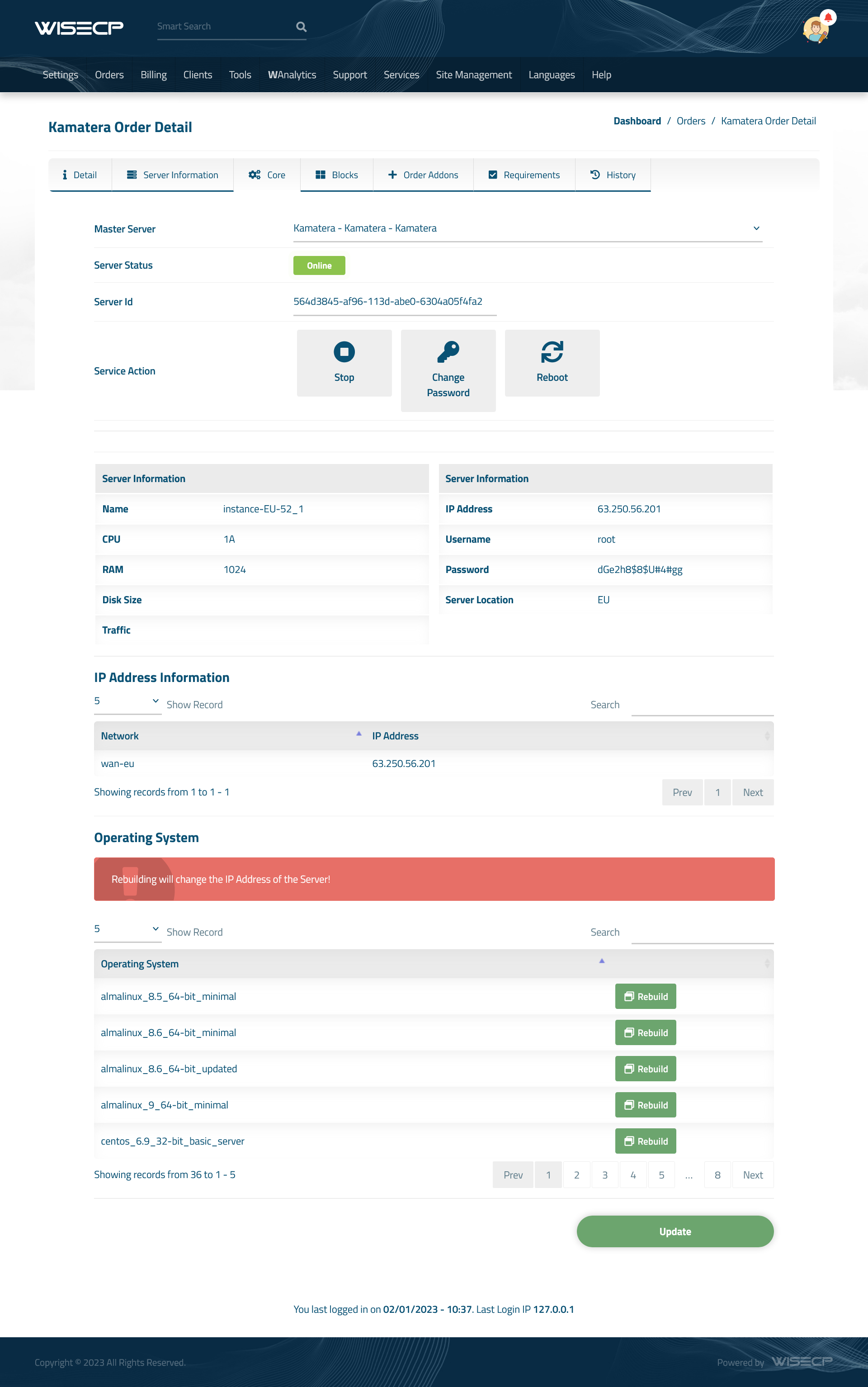**Image Caption: Detailed Interface of the Wyssep Website - Kamatera Order Detail Page**

This image showcases the user interface of the Wyssep website, characterized by a clean, white background with blue accents. At the top left of the page, the company name "Wyssep" is prominently displayed. Below this, a navigation bar presents multiple menu options including Settings, Orders, Billing, Clients, Tools, W, Analytics, Support, Services, Site Management, Languages, and Help.

The focal point of the page is the "Kamatera Order Detail" section. On the right side, the breadcrumb trail reads "Dashboard > Orders > Kamatera Order Details."

Within the primary window are several tabs for navigation: Details, Server Information, Core (currently selected), Blocks, Order Add-ons, Requirements, and History. The "Core" tab details are as follows:

- **Master Server**
  - Server Status
  - Server ID: Information displayed accordingly

Below, operational actions are presented with options to Stop, Change Password, or Reboot the server.

Two additional windows under the core information:
1. **First Server Information Panel**:
   - Name
   - CPU
   - RAM
   - Disk Size
   - Traffic

2. **Second Server Information Panel**:
   - IP Address (displayed prominently)
   - Username
   - Password
   - Server Location

Below the IP address details, a significant red warning informs: "Rebuilding will change the IP address of the server." Subsequently, a list of available operating systems is shown alongside a green "Rebuild" button.

Towards the bottom right corner of the screen is an "Update" button for any changes made on the page.